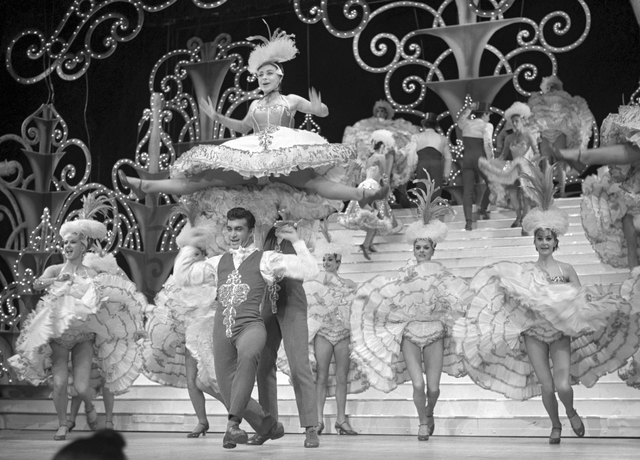This black and white image, resembling an old-style photograph or scene from an MGM musical, captures a vibrant and glamorous performance evoking the grandeur of a Las Vegas or Atlantic City show. Center stage is a man, reminiscent of Ricky Ricardo from the Lucy show, dressed in an embroidered vest and puffy shirt that blends seamlessly into his pants, energetically dancing. Surrounding him is a dazzling array of showgirls adorned in big, flowing skirts and elaborate feathered headdresses. Many of the women are engaged in a lively can-can type of dance, adding to the spectacle. One showgirl is dramatically lifted into the air behind him, showcasing the same voluminous skirt and headdress, enhancing the overall sense of movement and exuberance in this captivating scene.